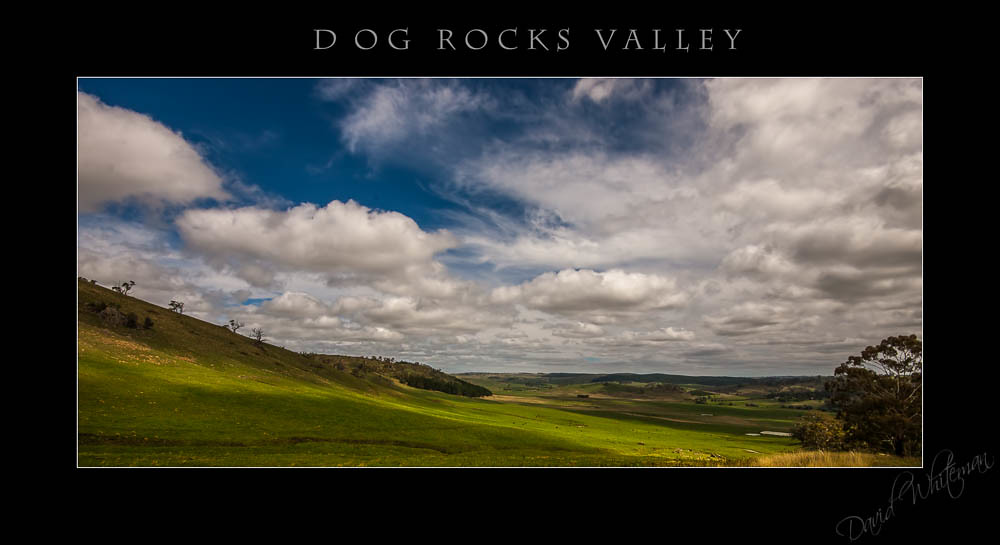The wide rectangular image, digitally framed with a black border and white inner lining, features the title "Dog Rocks Valley" at the top in thin white font. In the bottom left corner, a faintly gray diagonal signature can be noticed. This stunning landscape captures a lush, expansive valley that gently slopes downward into distant hills. The valley is predominantly a deep green, dotted with small plants, with a striking tall tree with green leaves situated in the bottom right corner. The sky dominates the upper portion, transitioning from a deep blue on the left to vibrant, thickly defined white clouds as it extends rightward. Small trees and other vegetation also pepper the hillside on the left, enhancing the natural beauty of the scene. The photograph masterfully captures the serene and inviting essence of Dog Rocks Valley.